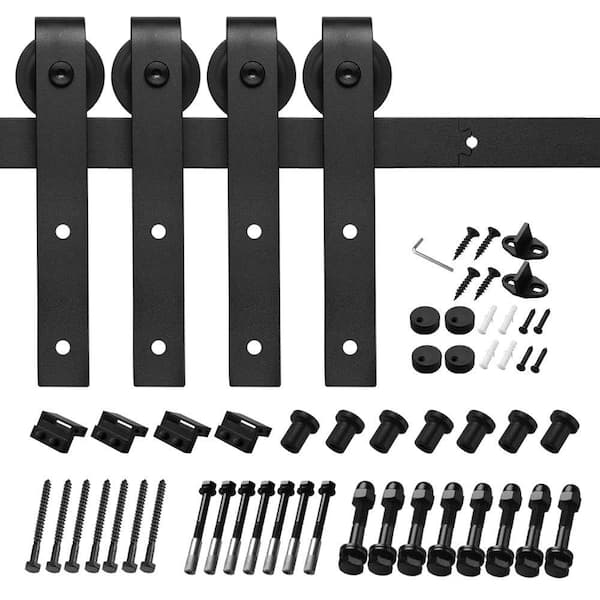The image appears to be a detailed layout of parts and hardware for assembling a sliding door system, likely for a barn or similar structure. Central to the image is a horizontal black or dark gray metal rail, approximately two inches wide and very thin, likely around 1/16 of an inch thick. On top of this rail are four sliding mechanisms consisting of brackets with built-in wheels, each featuring two bolt holes for mounting.

Surrounding the central rail and sliders is an array of assorted hardware grouped by type, including:

- An Allen wrench (hex key) to the right of the rail.
- Four screws, each paired with an anchor, and another set of four standalone screws.
- Two black brackets and four anchor screws.
- Multiple bolts paired with lug nuts, categorized into sets of eight.
- Several black circular discs with holes, likely used for securing the bolts.
- Various other sets of screws and pins, including eight short black pins and an equal number of nail-like screws.

The arrangement is highly organized, with each type of hardware neatly placed together, emphasizing the comprehensive assortment necessary for the installation of the rail and its components.